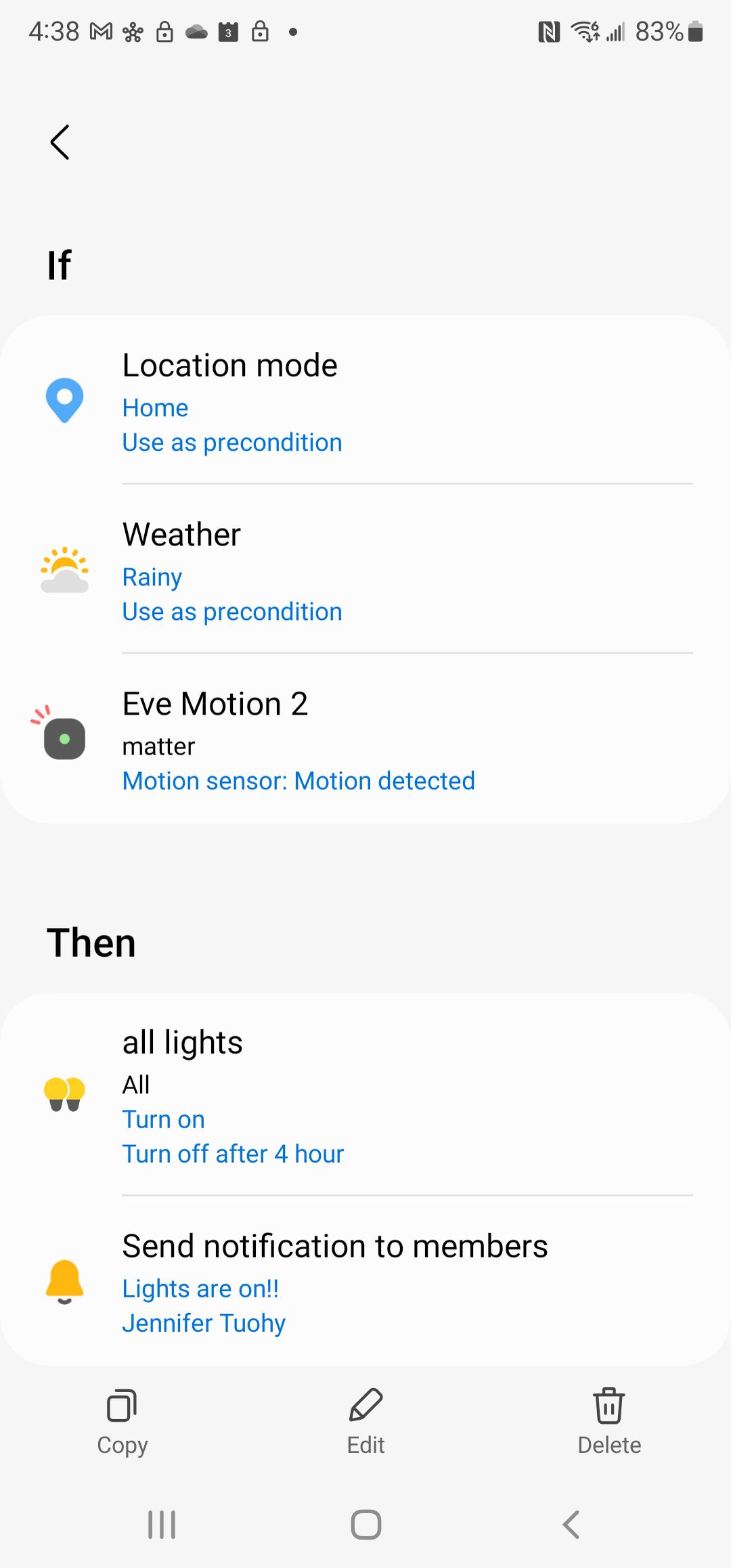In the image, there is a light blue background. At the top of the screen, the status bar displays "4:38" on the left, the battery level at "83%" on the right, and various icons including a leftward arrow. Below the status bar, the text "If" is prominently displayed.

Following this, there is a box labeled "Location Mode" featuring a small blue pin icon. This box displays the text "Home" and notes that it "Uses Precondition."

Next, another box labeled "Weather" with an icon depicting rain. This box displays the information "Rainy" and also indicates that it "Uses Precondition."

Below that is a section titled "Ease Motion 2,” specified as associated with a motion sensor. The phrase "Motion Detected" accompanies this section.

Subsequently, a small blue box contains the word "Then," indicating subsequent actions.

Directly following this cue, there is a box labeled "All Lights" which details that "All turn on" and "Turn off after 4 hours."

Another box states the action to "Send Notification to Members," with the message "Lights are on" directed to the user "Jennifer Touche."

At the bottom of the screen, there is a blue box with options labeled "Copy," "Edit," and "Delete." This section also includes icons for a menu with three lines, a square, and a left-facing arrow.